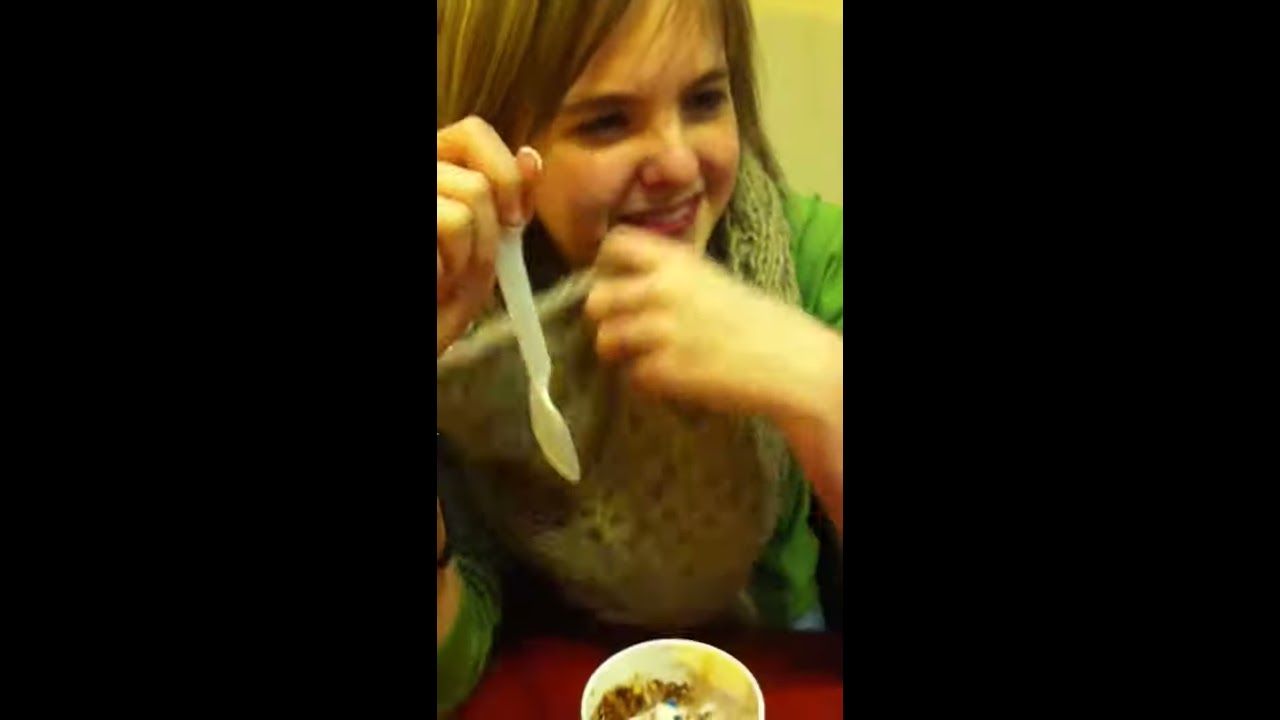This candid, low to medium quality photograph depicts a woman with light brown hair and a French manicure eating a dessert, likely ice cream or yogurt, using a white plastic spoon in her right hand. The woman, dressed in a green shirt and a fine gray knitted scarf, is sitting at a red table in a room with yellow walls. She is smiling and looking at someone out of frame, suggesting she's engaged in a pleasant conversation. Her left hand is clutched near her face as she enjoys her treat, which is almost finished. Although the image is slightly blurry and artificially lit, it captures her cheerful demeanor and warm interaction amid a casual dining setting. The photograph is bordered by two-inch vertical black panels on the left and right, emphasizing the central positioning of the woman.